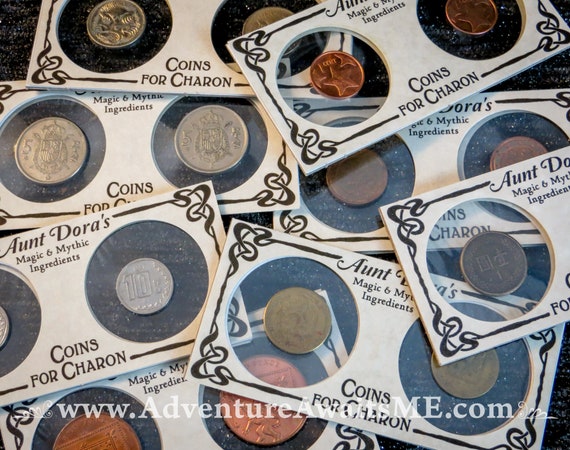Displayed in the image is a collection of collectible coin holders, meticulously designed and laid out on a black background. Each holder is rectangular, resembling the dimensions of dollar bills, and crafted from what appears to be printed cardboard, adorned with intricate black scrollwork patterns along the borders, lending a fancy and vintage aesthetic. Within each holder are two coins, enclosed in transparent circular plastic windows. The coins range in appearance, featuring silver, copper, dull brass, and bronze hues, with varied imprints such as stars and numbers, suggesting their special edition or collector's item status.

At the very top of each holder, in prominent black print, is the heading "Aunt Dora's Magic and Mythic Ingredients," with a subheading below it that reads "Coins for Charon" (stylized as "Coins for CHARON"). The bottom of each holder bears the watermark "www.adventureawaitsme.com," also rendered in white text. The holders exhibit a sense of cohesion and uniformity, reflective of an ornate and curated collection designed to captivate enthusiasts of mystical and mythical memorabilia.